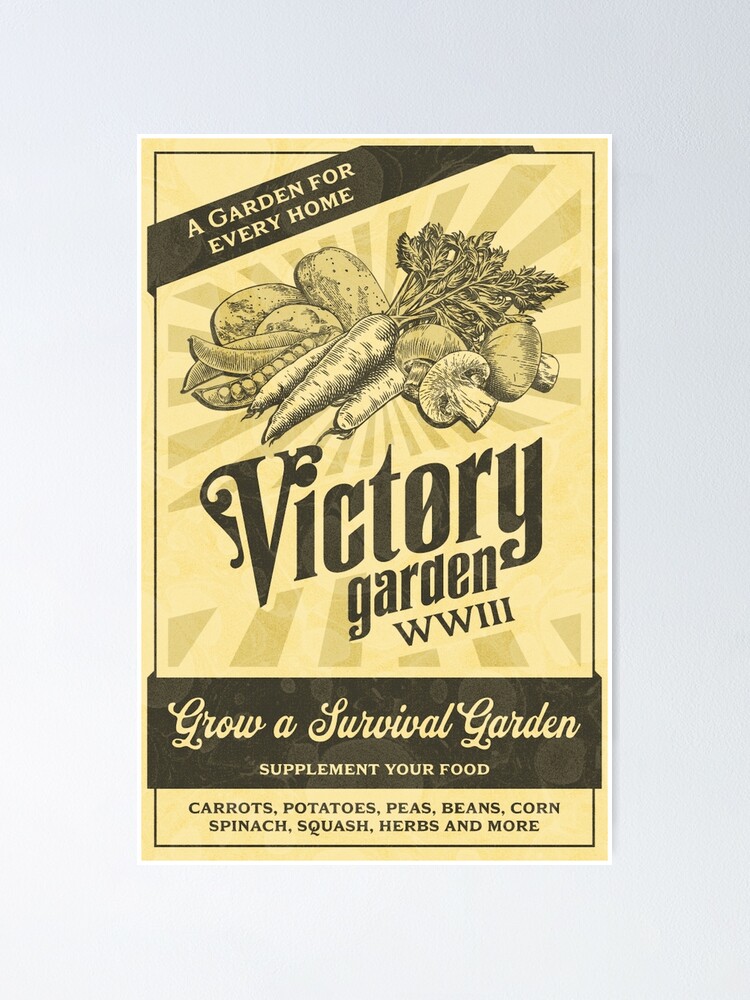This is a photograph of a vintage book cover with a sepia-toned background featuring an intricate sketch of various vegetables, including carrots with their stems, portobello and white mushrooms, green peas, potatoes, and squash. The top left corner of the cover displays a diagonal black banner with the phrase "A Garden for Every Home" in white script. Below the illustrations, bold black letters declare "Victory Garden, World War III." The lower portion of the cover has another black banner that reads "Grow a Survival Garden, Supplement Your Food" in elegant script, followed by a list of vegetables: carrots, potatoes, peas, beans, corn, spinach, squash, herbs, and more. Adding to the vintage feel, rays reminiscent of sunbeams radiate behind the vegetable illustrations, giving the entire cover a nostalgic and motivational aura.